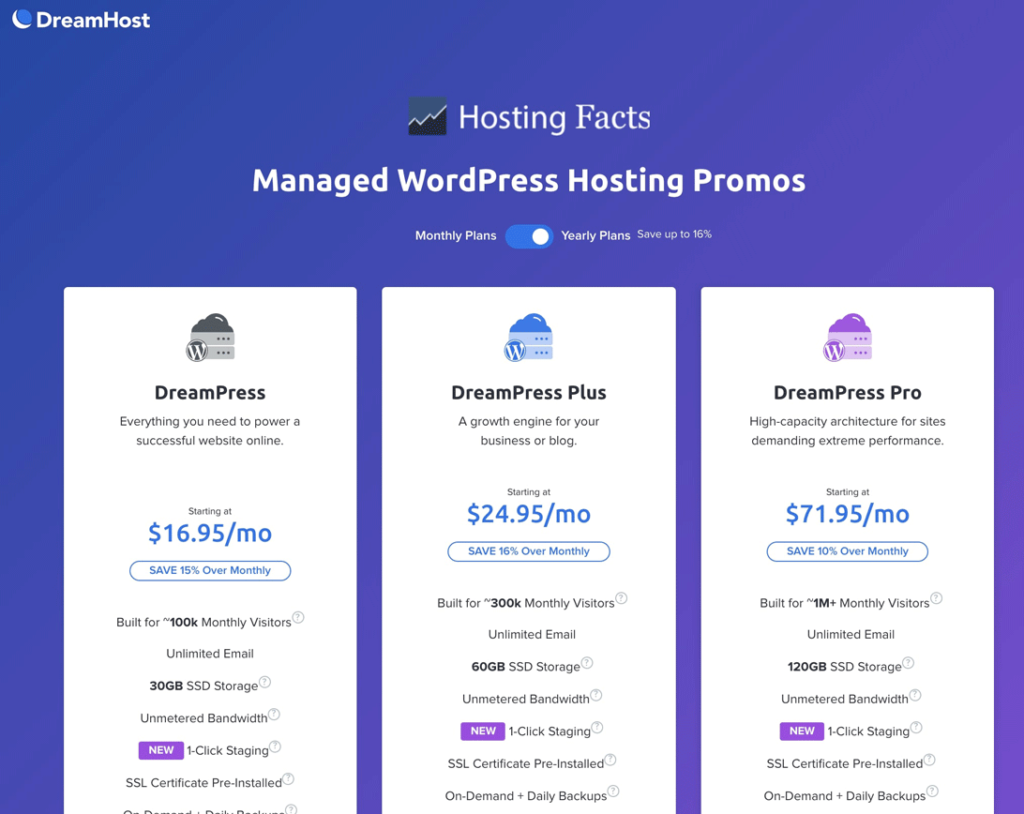The image is a screenshot of what appears to be a computer screen, featuring a Dream Host page. In the upper left-hand corner, the "Dream Host" logo is prominently displayed. The central section of the screen header is titled "Hosting Facts," followed by "Managed WordPress Hosting Promos," along with options for "Monthly Plans" and "Yearly Plans." A toggle bar is present between these two options, with the setting currently set to "Yearly Plans." 

The text highlights a promotional offer for yearly plans, stating "save up to 16%." 

Below this section, three rectangular boxes are laid out horizontally, each detailing a different version of DreamPress hosting plans:

1. **DreamPress:**
   - Description: Everything you need to power a successful website online.
   - Price: Starting at $16.95 a month (saving 15% over monthly rates).
   - Features: Support for 100,000 monthly visitors, unlimited email, 30 GB SSD storage, unmetered bandwidth, new one-click staging, and a pre-installed SSL certificate. Additional details are cut off in the image.

2. **DreamPress Plus:**
   - Description: A growth engine for your business or blog.
   - Price: Starting at $24.95 a month (saving 16% over monthly rates).
   - Features: Support for 300,000 monthly visitors, unlimited email, 60 GB SSD storage, unmetered bandwidth, new one-click staging, a pre-installed SSL certificate, and on-demand plus daily backups.

3. **DreamPress Pro:**
   - Description: High capacity architecture for sites demanding extreme performance.
   - Price: Starting at $71.95 a month (saving 10% over monthly rates).
   - Features: Support for 1 million+ monthly visitors, unlimited email, 120 GB SSD storage, unmetered bandwidth, new one-click staging, a pre-installed SSL certificate, and on-demand plus daily backups.

Overall, the image provides a comparative overview of different DreamPress hosting plans, emphasizing their unique features and promotional pricing for yearly subscriptions.